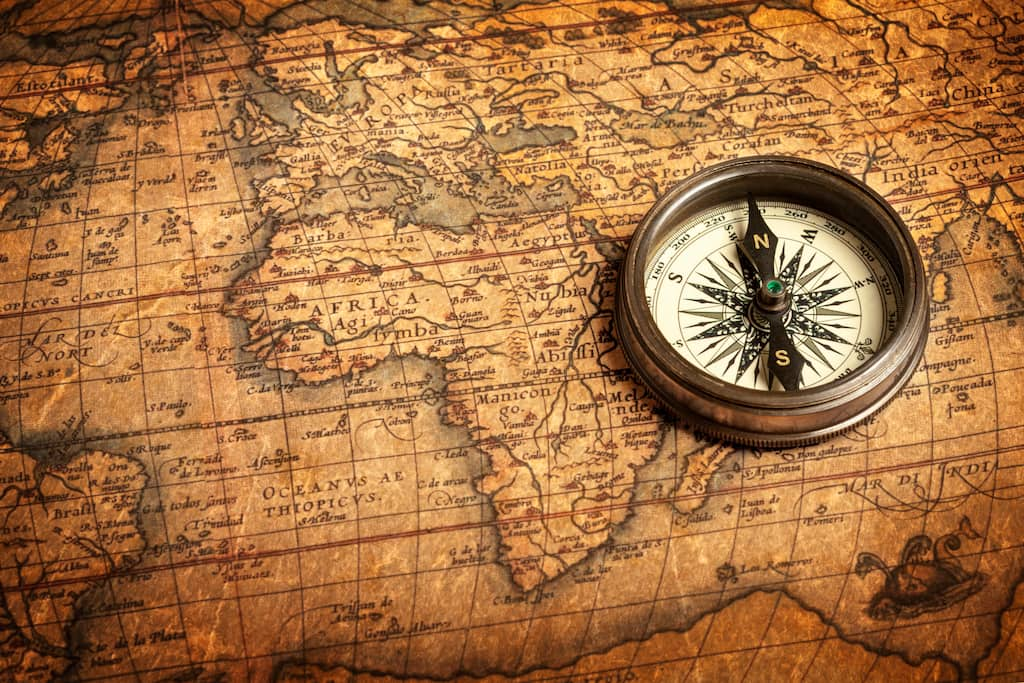The photograph captures a detailed scene of a small, round weathered brass compass resting on an old-style map. The map, which seems to be drawn on parchment paper, is centered over the continents of Africa, Europe (labeled as "Europa" with a "V" instead of "U"), and parts of Asia. The map is richly detailed with black grid lines and various place names in Latin, such as "Tartaria" and "India Orientalis." Sea monsters and other classic cartographic elements adorn the oceanic spaces. The compass, positioned on the right side of the map, has a white face with black heading numbers and lines indicating degrees and cardinal directions. The north arrow is marked with a brown "N" and points between west and south, while the south arrow has a brown "S." The ring of the compass itself is oriented towards the southwest. The map’s faded, hand-drawn appearance contrasts sharply with the sharp, purposeful design of the compass, merging an explorer's tools with the spirit of ancient cartography.